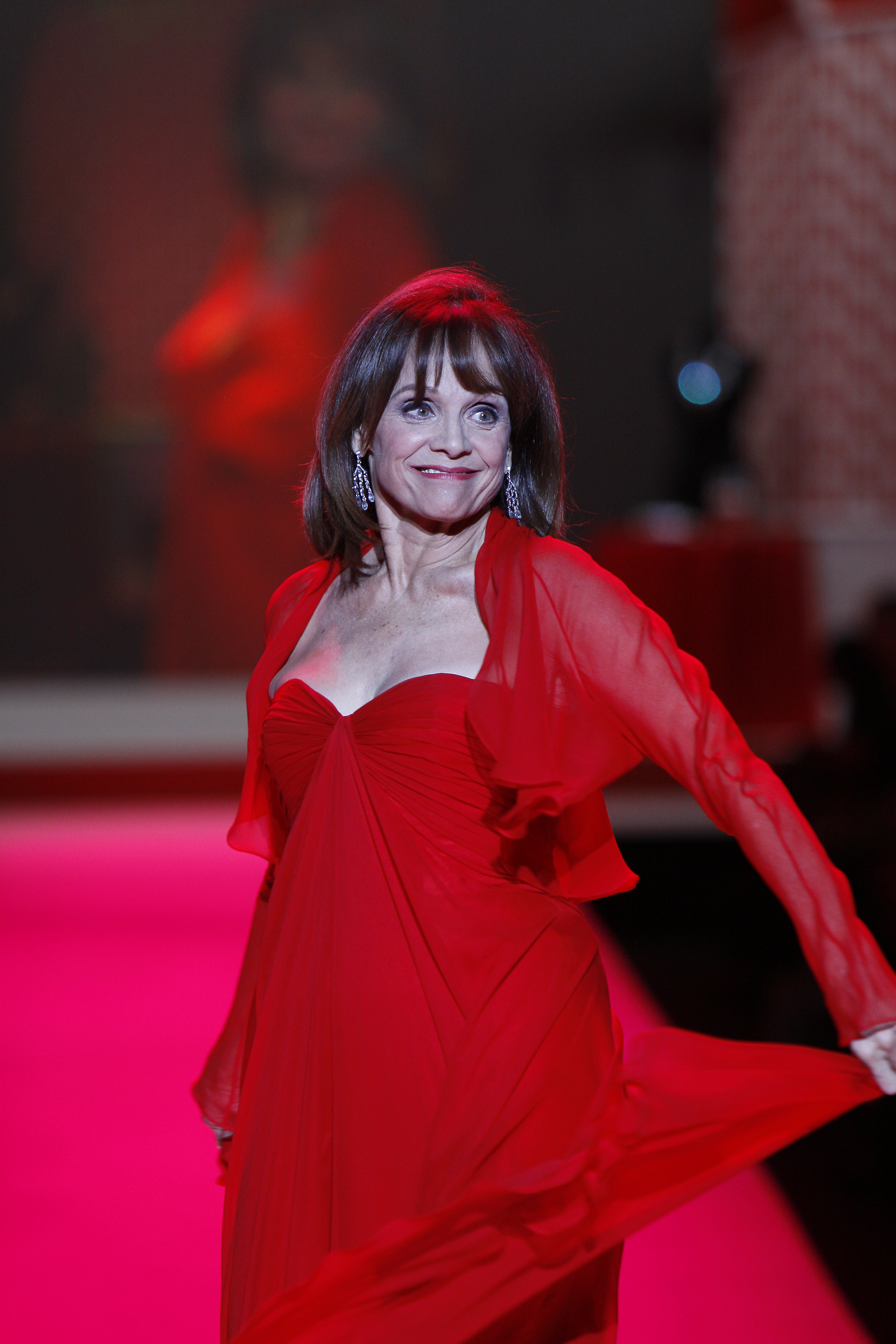The photograph depicts an older Caucasian woman, likely in her late 60s, standing on what appears to be a red carpet or runway, possibly during a fashion show. The woman is dressed in a striking red dress featuring a sweetheart neckline and ruching around the chest area. She accessorizes with a sheer, waist-length red cape, which is see-through and opened in the front. Her left hand (right from the viewer’s perspective) is holding out part of her flowing skirt. 

She has shoulder-length black hair with bangs and is adorned with silver chandelier earrings. Her makeup includes vibrant red lipstick. The expression on her face reveals a slight grimace, showing her teeth on the left side of her mouth while the right side remains closed.

In the background, there is a blurred projection of the woman herself, adding a sense of depth and repetition to the scene. The stage or carpet she is on is highlighted in pink tones. Additionally, a distinct white strip horizontally crosses the middle of the image, intersected by a smaller red strip, with a blue light beam directed towards her, illuminating her presence further.